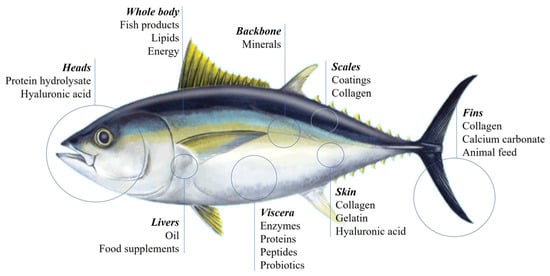The image is an anatomically detailed illustration of a tuna on a white background, showcasing various color gradients and precisely labeled parts of the fish. The fish is depicted with a blue stripe on top, a lighter blue stripe beneath, then a greenish-yellow stripe, and a white belly. The top fin near its head is yellow, while the middle fin is a mix of gray and white, and the tail fin is also blue with yellow spikes around it. 

Each part of the fish is labeled with circles and lines pointing to the specific areas, and these labels include the head, whole body, backbone, scales, fins, skin, viscera, and liver. Below each labeled part, there are further detailed descriptions. For example, the head is marked with "Heads," followed by "protein, hydrolysate, hyaluronic acid." The whole body is labeled with "Fish products, lipids, energy," while the backbone is annotated with "Minerals." The scales are indicated with "Coating, collagen," the fins with "Collagen, calcium, carbonate, animal feed," the skin with "Collagen, gelatin, hyaluronic acid," the viscera with "Enzymes, proteins, peptides, probiotics," and the liver with "Oil, food supplements." 

This precise and detailed annotation provides a comprehensive overview of the various components and potential uses of each part of the fish.